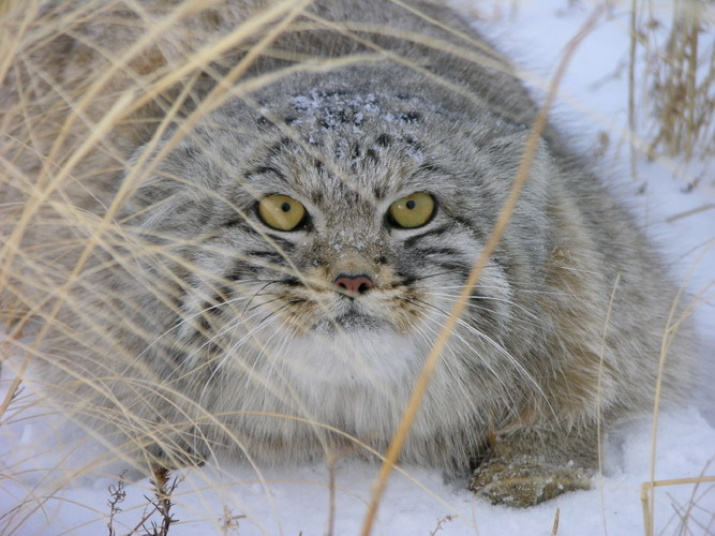This captivating wildlife photograph features a small wild cat lying on its stomach in the snow, directly gazing into the camera with its mesmerizing, big yellow eyes, which hold a central black pupil. The cat's fur is a striking mix of gray, white, and black, thickest between its eyes and up its forehead. A light layer of snow delicately rests on its head, and its ears are laid back, contributing to its alert appearance. Its face exhibits a beautiful contrast, with a light orange and black-trimmed nose above a brown-tinted muzzle. The cat's whiskers are a blend of black and white, gracefully extending from its face. The fur transitions from white under the chin to gray further down the body. The background and surroundings of the image consist of dried, brown grass peeking out from the blanket of snow, creating a stark contrast that highlights the cat's intricate fur pattern. Despite the limited color palette of white, brown, gray, and black, the cat's piercing eyes dominate the composition, making it a striking image suitable for a wildlife setting or website.